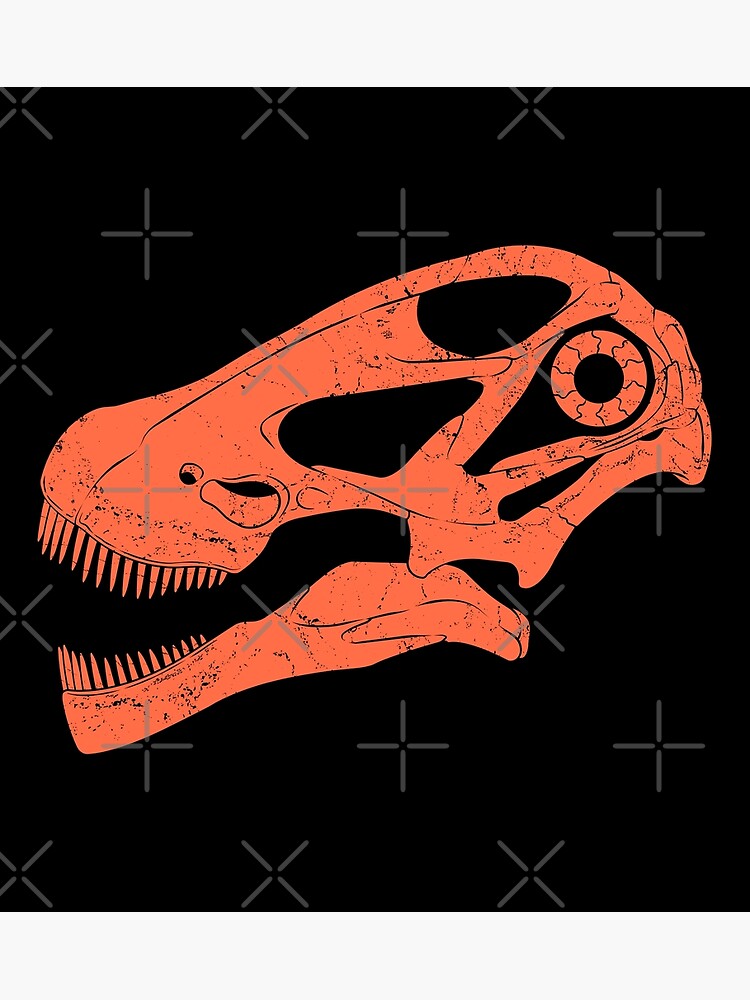The image features a digital or painted depiction of an unidentified animal skull, which could likely belong to a dinosaur or another carnivorous predator, indicated by its numerous sharp teeth. The skull, which is predominantly a fluorescent orange or peachy color, has an oval-shaped structure with a rounded snout and a flat jawline. It also contains black specks and empty spaces where eyes might have been. The background is a plain black canvas adorned with a pattern of light gray X's and crosses stretched from the top to the bottom. Additionally, there is a peculiar, large circular feature in the top right part of the skull, marked by a black center surrounded by an orange ring with radiating squiggly lines, possibly suggesting an eye socket.